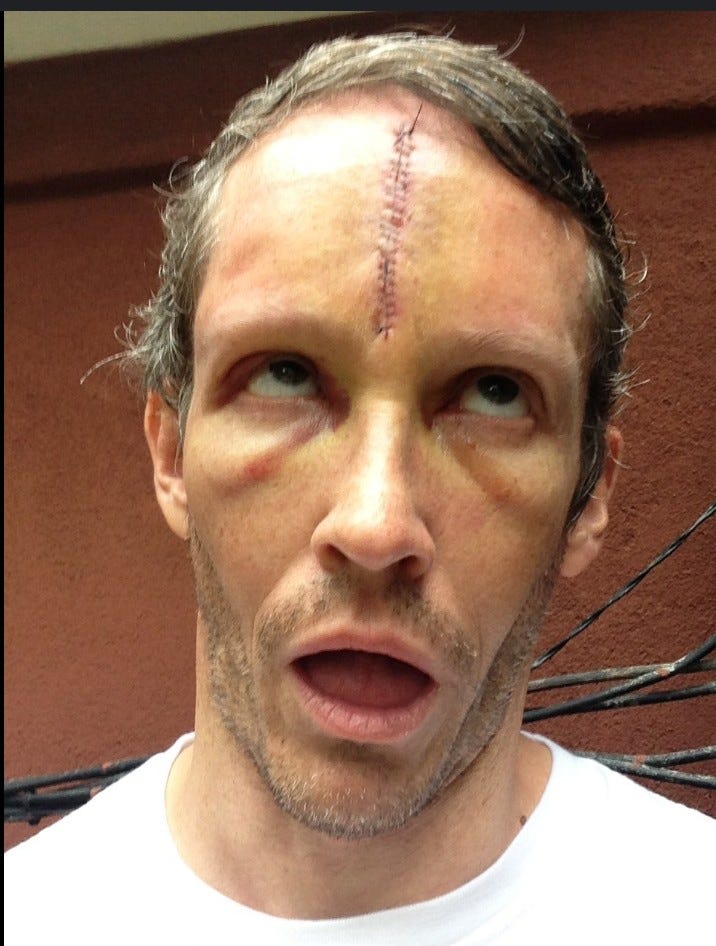This detailed close-up photograph captures a white male with short brown hair, standing against an orange wall accented with black cables and wires. His facial expression is one of lost contemplation, as his mouth hangs open and his eyes gaze skyward. Prominently, a long vertical scar, complete with red stitches, runs from the top of the bridge of his nose to his hairline, suggesting recent surgery. His face shows signs of fatigue, with noticeable bruising and bags under his eyes. The man sports a scrubby beard, indicative of not having shaved for several days, and he's dressed in a white t-shirt. The lighting and composition of the image emphasize the dramatic and possibly introspective nature of his demeanor.